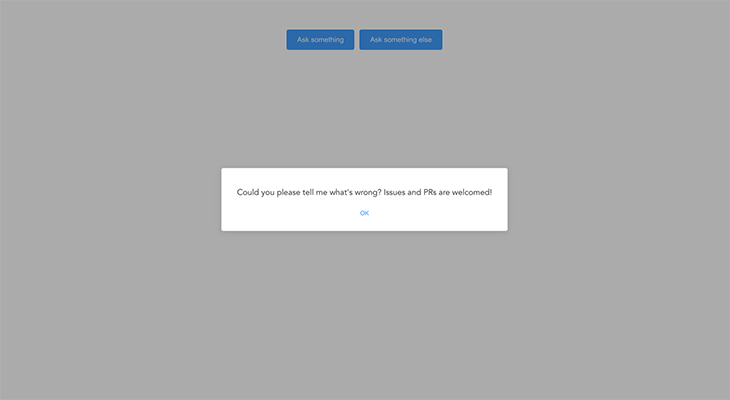A screenshot of a grayed-out webpage features a prominent white, rectangular pop-up box in the center with the message, "Could you please tell me what's wrong? Issues and PRs are welcomed!" The message is concluded with an exclamation mark for emphasis. Below the text, there's an "OK" option displayed in blue text. In the blurred background surrounding the pop-up, two additional rectangular blue buttons are visible. The first button reads, "Ask Something," and the second button reads, "Ask Something Else." The composition captures a clear focus on the user prompt, indicating an interactive element seeking user feedback.